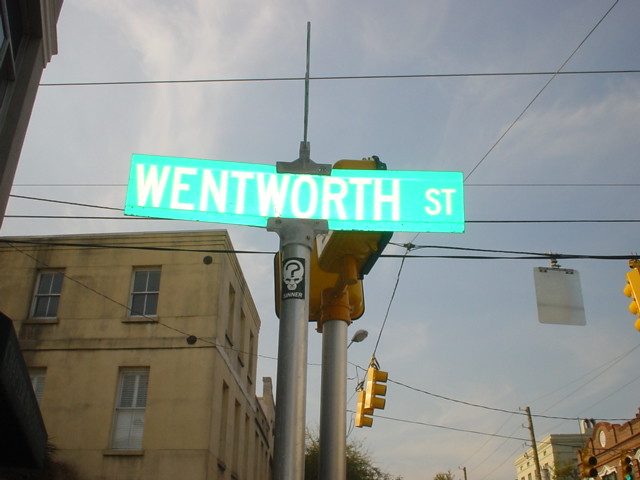In this landscape photograph, a bright green street sign reading "WENTWORTH STREET" in white capital letters is prominently displayed in the center. The sign, mounted on a round silver metal pole adorned with a small black sticker depicting a white skull, reflects light possibly from a camera flash. Surrounding the sign are several noteworthy elements: a yellow traffic light with a silver metal pole visible behind the street sign, and another hanging traffic light with its yellow back. The scene is set against a blue sky with wispy white clouds, featuring multiple electrical and hydro wires. To the right of the sign, there are beige and brown multi-story buildings, and to the left, a beige brick building with dark-colored windows. A faded yellow building appears in the bottom left of the image, while a building with a red roof is seen in the bottom right. Sparse trees are also visible in the background, adding to the urban landscape.